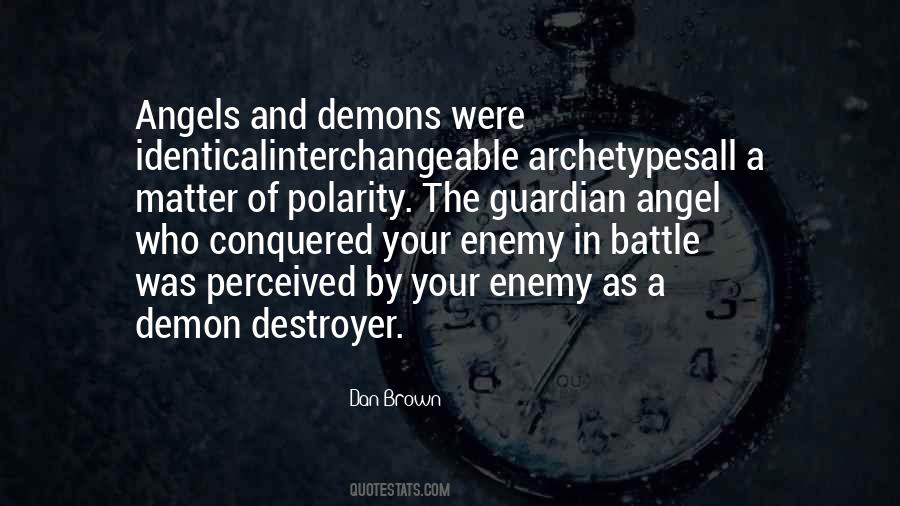The image showcases a paragraph of white text on a dark background. The text reads: "Angels and demons were identical, interchangeable, archetypes, all a matter of polarity. The guardian angel who conquered your enemy in battle was perceived by your enemy as a demon destroyer." Below this quote, the name "Ben Brown" and the URL "ColdStats.com" appear in smaller font. The background features an old circular clock with a black rim and a worn white face, indicating the time as 5:35. The numbers around the clock are in a Western numeral format, with some of them appearing faded. The clock is positioned towards the center-right part of the image, slightly blended into the dark background. The quote is left-aligned but fairly centered horizontally within the image.